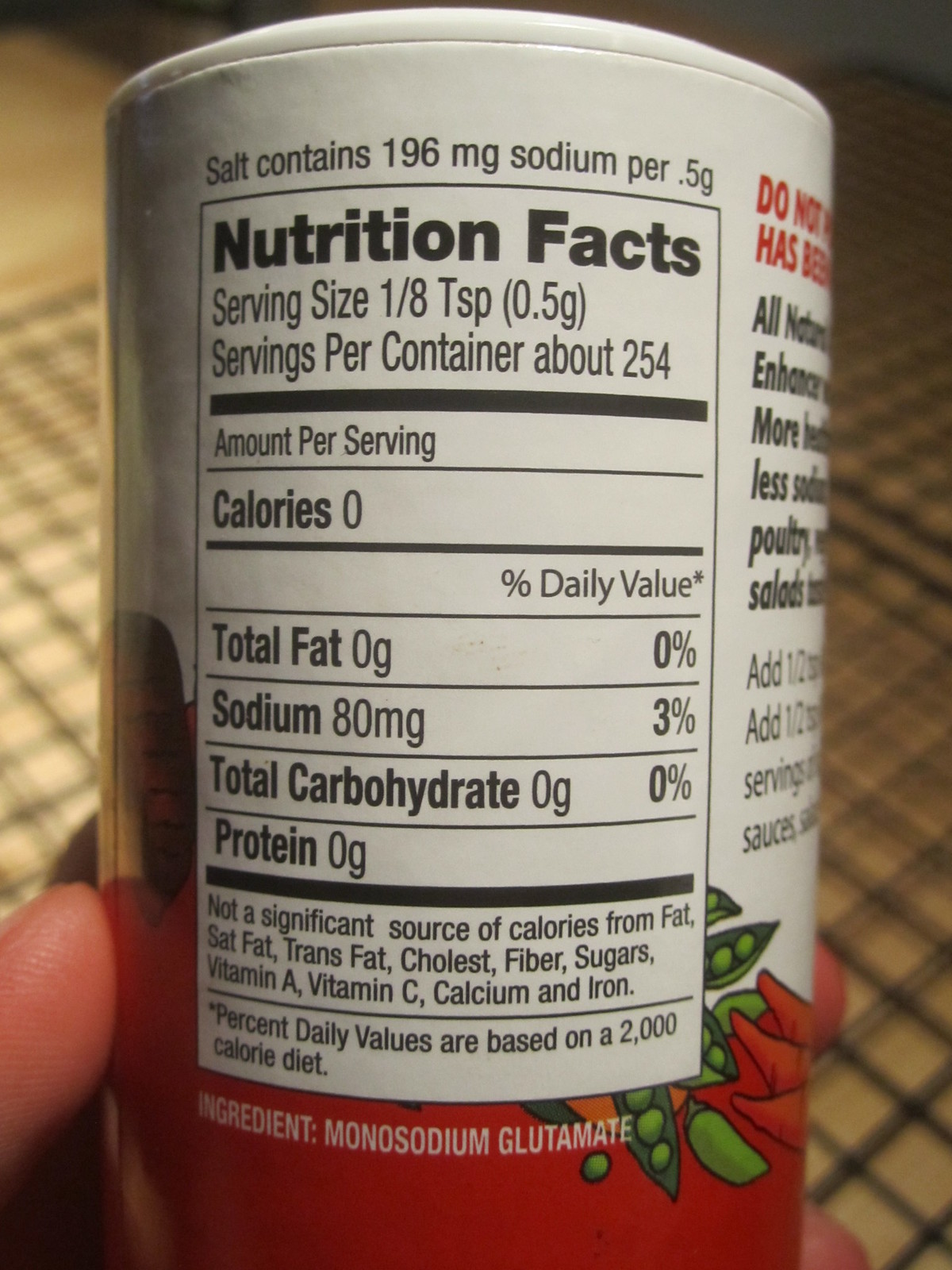The image shows a small, white container of monosodium glutamate seasoning, commonly known as MSG. The container features a red base and displays a graphic of assorted vegetables on the front. The back of the container provides detailed nutritional information: it contains 196 milligrams of sodium per 5 grams, equating to 80 milligrams of sodium per serving, which is 1/8 teaspoon. Each serving represents 3% of the recommended daily value for sodium. The container holds approximately 254 servings. The nutritional facts indicate that it has zero calories, no total fat, no total carbohydrates, and no protein. Additional text on the container notes that it is not a significant source of calories from fat.